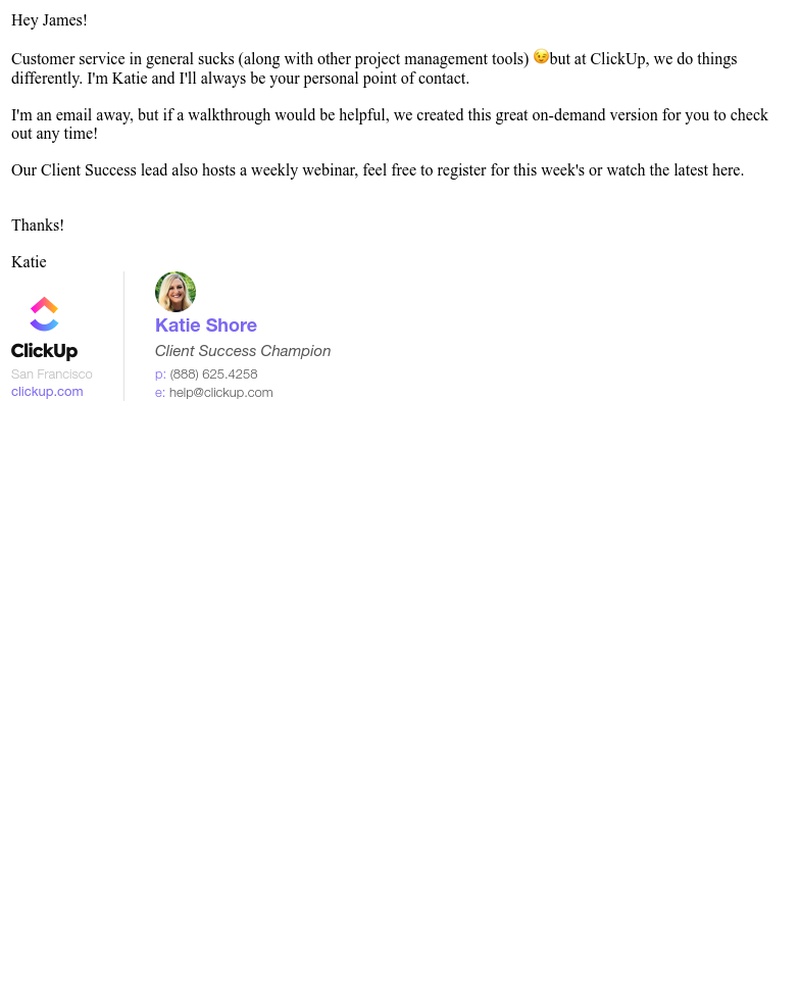In this image, a professionally dressed man, identified as James, is reading a message from Katie Shaw, who is a Client Success Champion at ClickUp. The message addresses common frustrations with customer service and project management tools, highlighting ClickUp's commitment to providing exceptional support. Katie introduces herself as James' personal point of contact, available via email for any queries or support. She also mentions an on-demand walkthrough created for users' convenience and invites James to register for weekly webinars hosted by their Client Success Lead. Contact details are provided for further assistance: 888-625-4258 and help@ClickUp.com. The ClickUp brand and Katie Shaw’s role are prominently featured at the end of the message.